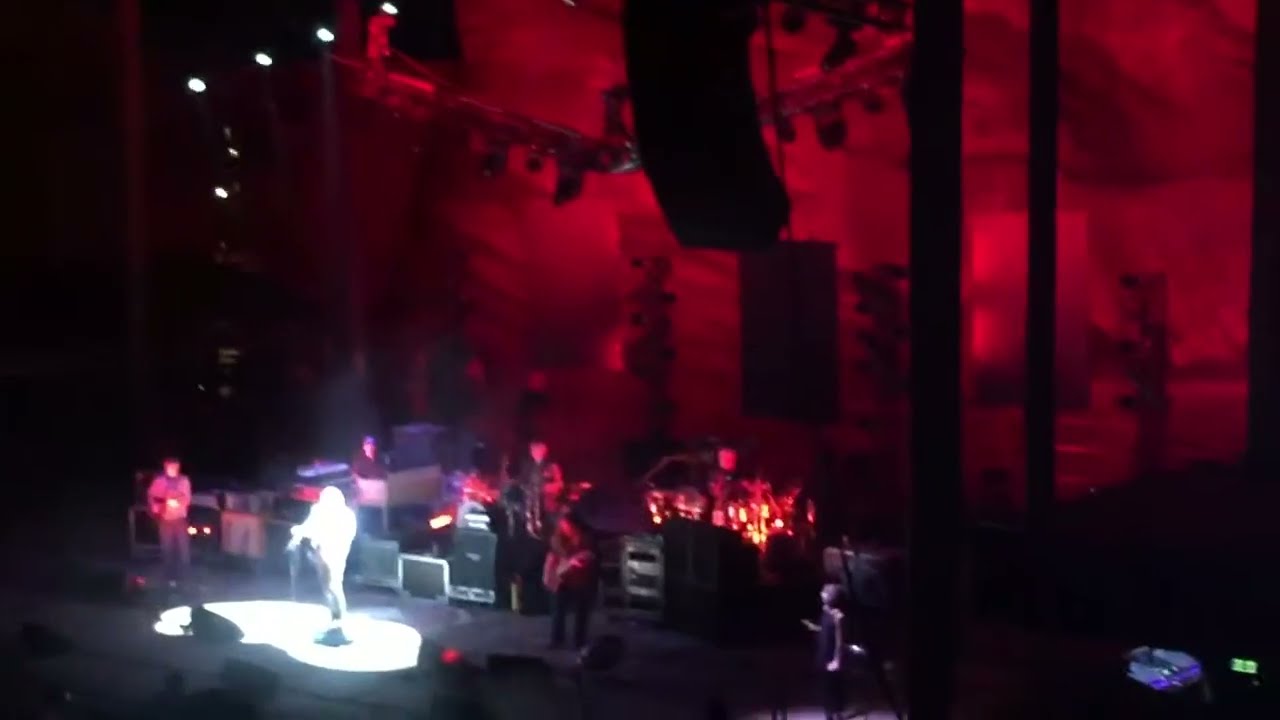The photograph captures a dynamic concert scene from an elevated vantage point, roughly 10 to 20 feet above the stage, centered on a rock band mid-performance. The lead singer, positioned in front of a microphone at the forefront of the stage, is completely washed out by an intense white spotlight, rendering them indistinguishable. Surrounding the lead singer, the stage is enveloped in a deep red glow that accentuates the other band members, including multiple guitarists and a drummer, who are partially visible despite the overall dimness. The background features a dark red wall interspersed with black vertical stripes and various rectangles, adding depth to the scene. Overhead, stage lights extend from the ceiling in the top left corner, casting directional beams down onto the performers. Black speakers, shaped like tall cubes, and other amplifying equipment are scattered behind the musicians, contributing to the atmosphere. The image, though blurry, vividly conveys the immersive and energetic ambiance of the live musical performance.